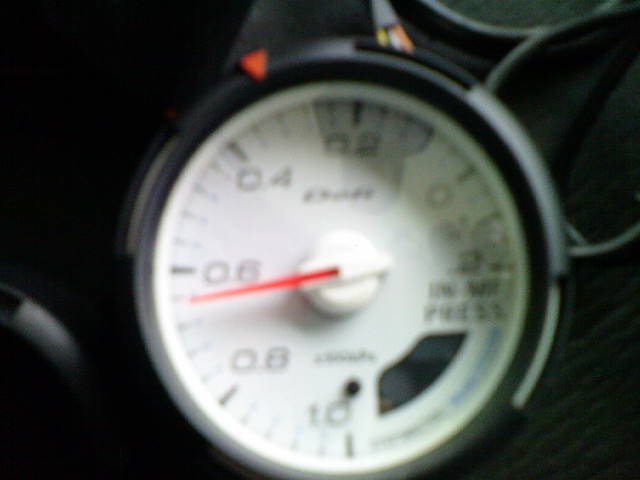This color photograph features a close-up shot of a pressure gauge. The primary focal point of the image is the gauge's face, which is white with bold black numerals. The scale ranges from 2 to 10, with numbers increasing in increments of two: 2, 4, 6, 8, and 10. The red needle on the gauge is pointing between the 6 and 8 marks, notably closer to 6. The photograph itself is somewhat blurry, obscuring finer details beyond the main features of the gauge.

The gauge's casing is black, providing a stark contrast to the white face. Surrounding the casing, one can see bits of metal and several wires connected to the gauge, although their destination remains unclear due to the image's tight framing. Despite the lack of clarity on external connections, it is evident that the gauge is functioning, as indicated by the needle's pointed position. This detailed shot encapsulates the essence of a working pressure gauge in operation.